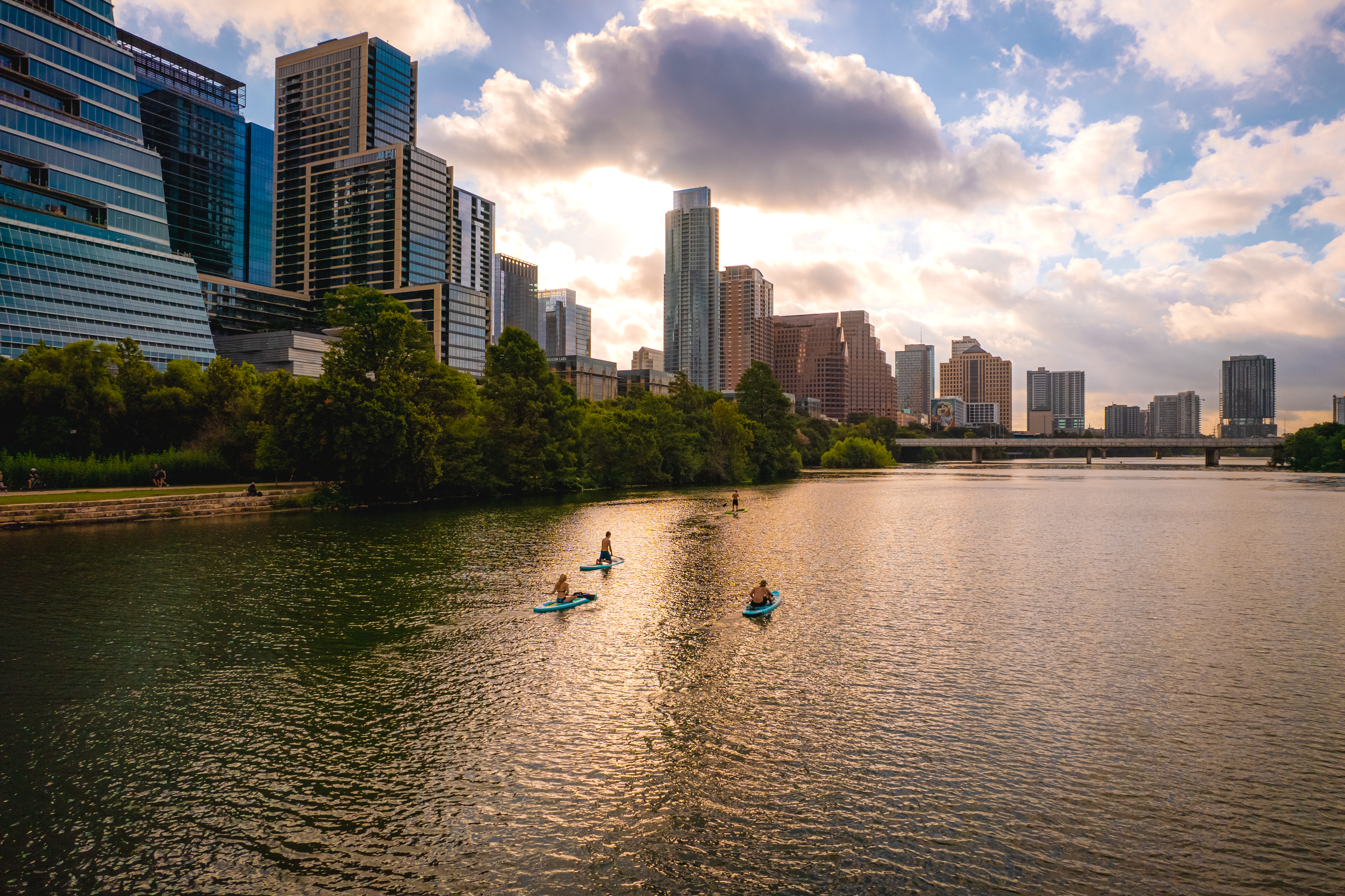The photograph captures a vibrant urban river scene on a sunny day amidst a modern cityscape. The river, approximately half a mile wide, is adorned with ripples, indicating a gentle breeze. Four individuals navigate the water in single-person aqua blue kayaks, each wearing life vests and paddling together toward the city. The left side of the river showcases towering skyscrapers with predominantly glass facades that reflect the light and the river’s surface. At the base of these buildings, a row of trees and a constructed wall can be seen lining the river’s edge. Additionally, a bridge spans the river in the distance, integrating seamlessly into the background of more tall buildings. The sky above is bright with large, fluffy clouds, and the sunlight piercing through reflects off the river, creating a harmonious interplay of reflections between the water and the city. Despite the occasional silhouette of distant figures, the primary focus remains on the quartet of kayakers exploring this urban waterway.